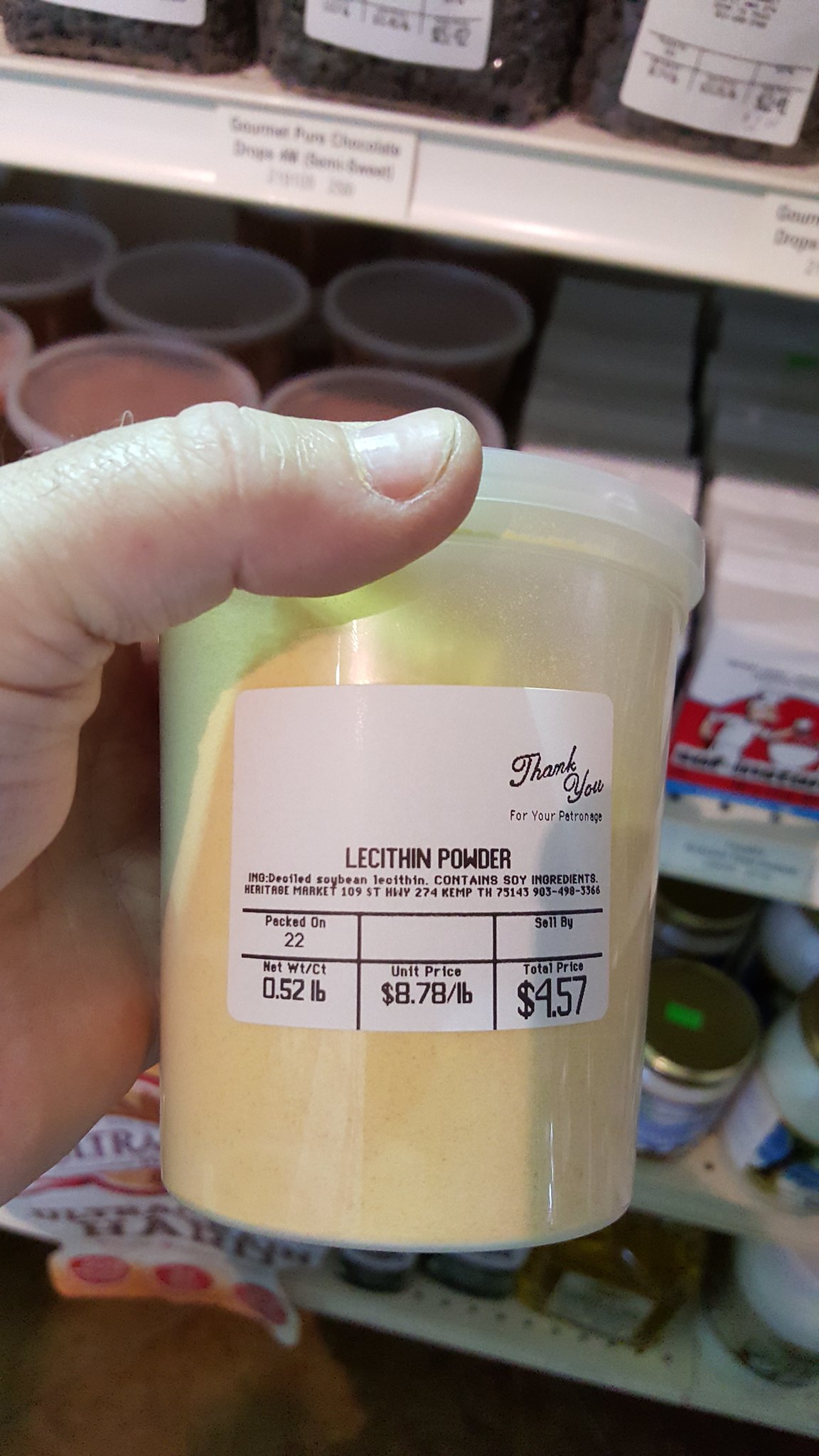This close-up photograph captures a plastic container being held by a person in a store. The white thumb of the individual is visibly placed on the top front of the container, while the fingers supporting it from the back remain out of view. The container, a small cylindrical vessel with a snap-on lid, weighs 0.52 pounds. The product label, though partially legible, prominently displays the words "LECITHIN powder." Below this, faint text mentions soy ingredients, though the details are unclear. Also on the label, there are six vertical rectangles with various information: the first specifies "packed on 22," the second is empty, the third notes "sell by" with no date provided, and subsequent lines indicate the net weight and pricing details. The unit price is set at $8.78 per pound, culminating in a total price of $4.57 for the item. The background of the image is blurred, showing additional store shelves lined with various indistinct products, reinforcing the retail setting.